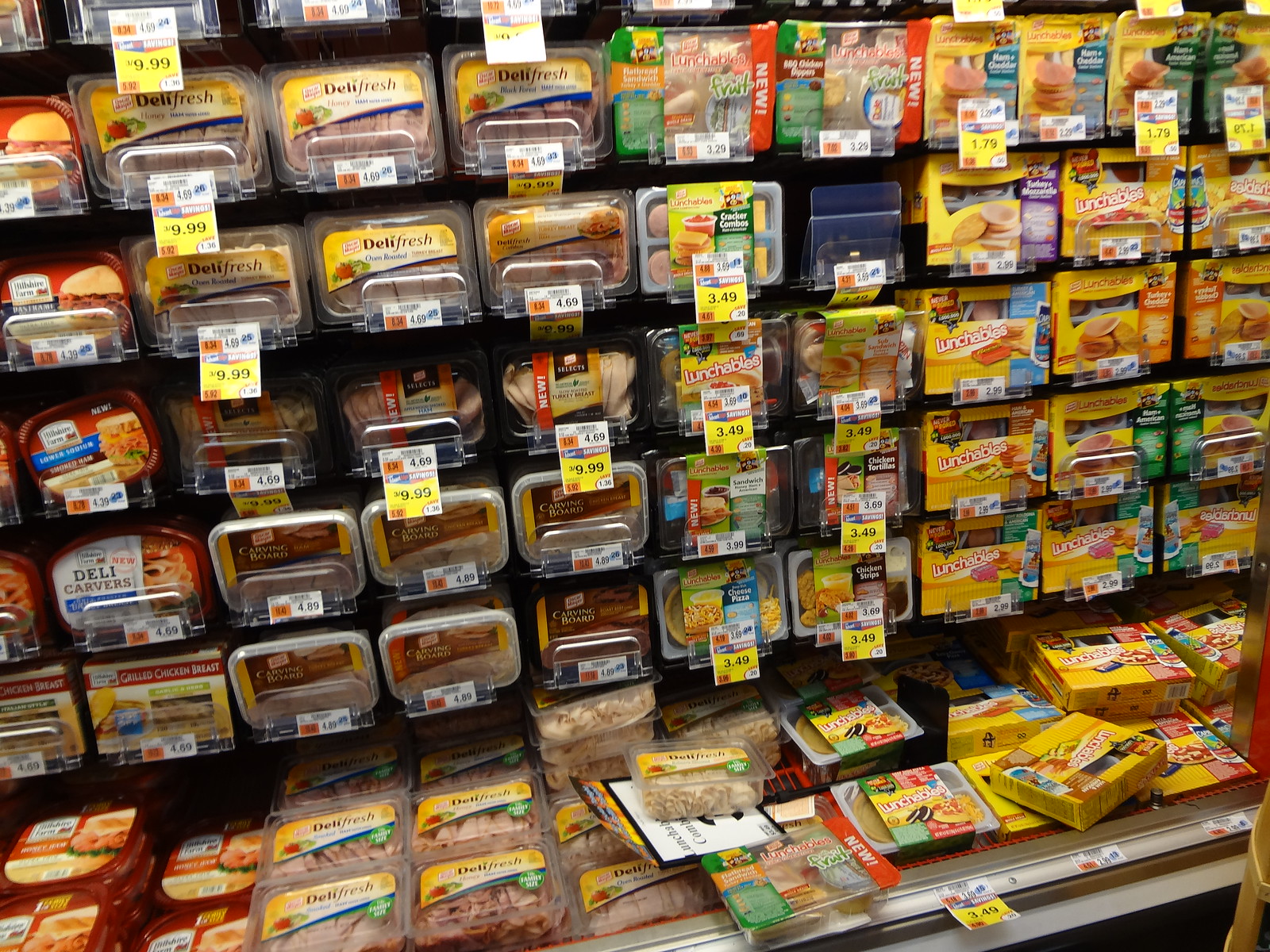This photo captures the deli meat section of a grocery store's cooler aisle, specifically designed for pre-packaged refrigerated foods without doors. The left side of the aisle is dedicated to a variety of sandwich meats, including popular brands like Hormel, Daily Carvers, Hillshire Farms, and Oscar Mayer, all neatly arranged in plastic clamshell packaging. The meat ranges in price, predominantly marked at $9.99 but becoming cheaper toward the right side, some as low as $4.69. On the right side, you'll find an assortment of Lunchables and similar meat, cheese, and cracker snack packs, with brands such as Daily Fresh. The displays are well-stocked except for one empty shelf. Each shelf features price tags, prominently displaying prices around $3.49 for some items. The overall setup is organized, with horizontally extending shelves of a gray or tan color, showcasing a wide variety of pre-packaged deli meat and snacks in rectangular packaging.